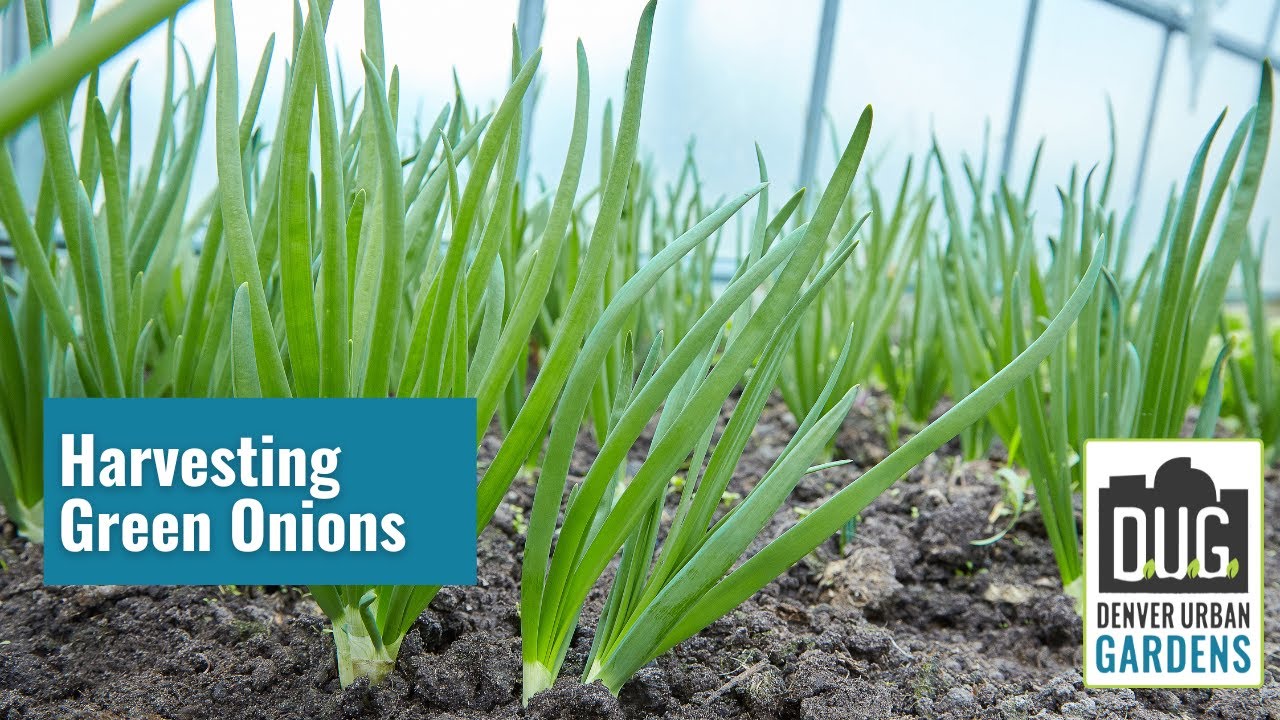This vertical rectangular image features a close-up view of green onions growing in soil. The soil appears dry and rugged, suggesting active tilling or a rough planting bed. The green onions are slender and predominantly green, with white bases emerging from the soil. The backdrop includes a partially visible fence with wide gaps, hinting at a garden space vulnerable to pests. Beyond the fence, a blue sky adorned with fluffy white clouds is visible. In the bottom left corner of the image, a blue rectangle contains white text reading "Harvesting Green Onions." The bottom right corner holds a white rectangle with the text "Denver Urban Gardens" and the acronym "DUG," where "DUG" is styled with little green leaves acting as separators. The photograph gives the impression of an urban garden setting, likely within a greenhouse, as suggested by the observed walls and meticulous planting.